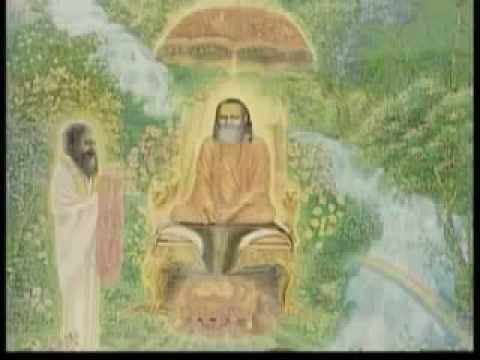The image depicts a detailed, older-looking piece of artwork with a stipple effect, possibly real or generated. The central focus of the image is a religious-style figure with a gray beard and dark, shoulder-length hair, seated cross-legged on a glowing golden throne. The throne, which has a fur draped over its seat and a foot cushion in front, is positioned under a large umbrella. The man is wearing an Indian-style robe, and he is situated in the center of the image. To his left, standing towards the bottom left corner, is another man dressed in white robes with black hair and a black beard, holding an object. They are both set in an outdoor, forested environment by the bank of a small blue stream, surrounded by lush green and yellow trees and flowers. The color palette includes green, white, gray, brown, black, orange, and yellow, contributing to the overall serene and pastoral atmosphere.